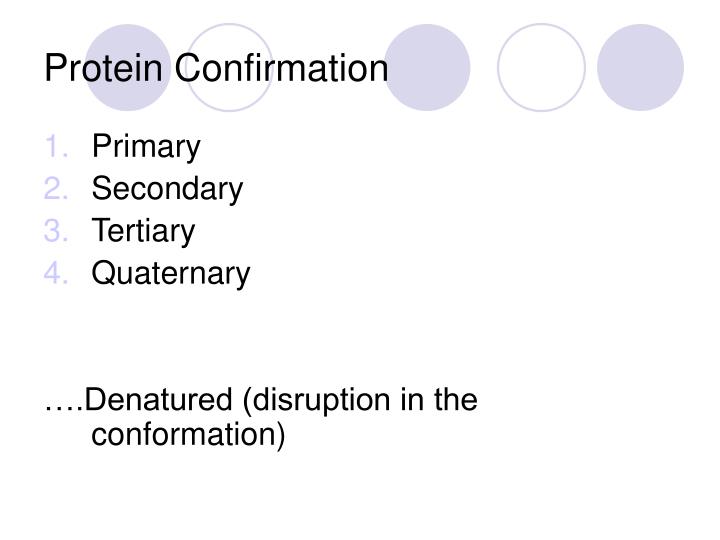The image features a white background with five circles aligned horizontally at the top. Three of these circles are light blue (or lavender purple), and two are white; they alternate colors and appear level. On the left side of the image, black text reads "Protein confirmation" followed by a numbered list in sequential order: "1. Primary  2. Secondary  3. Tertiary  4. Quaternary." Each number is written in a lighter color (lavender type of outline or grayed out). Below this list, the text continues with "... Disruption in the confirmation," indicating a denatured state. The text and numbers are primarily typed in a clear, black font.